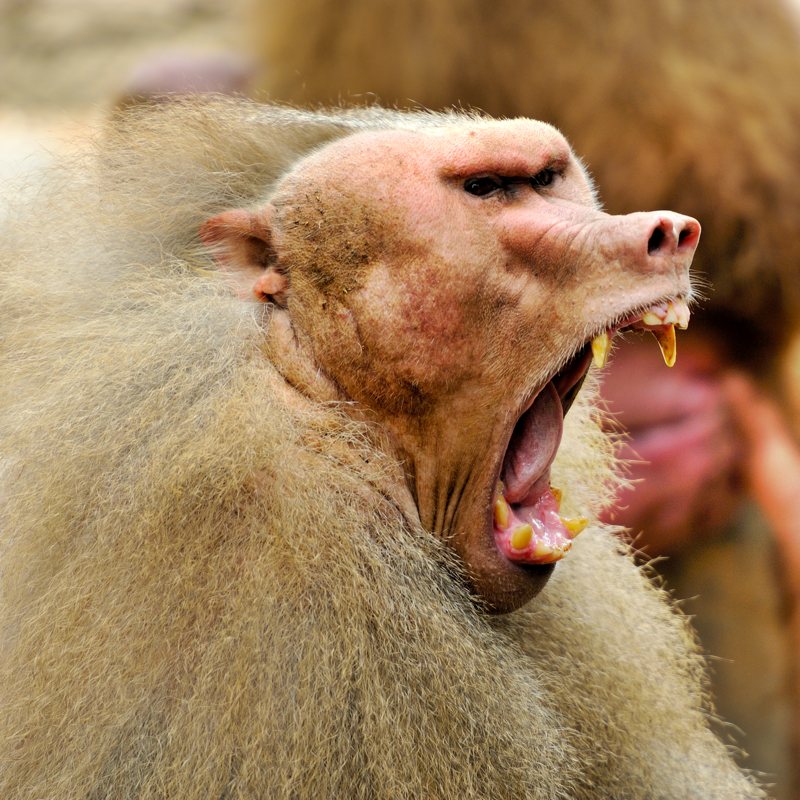In this detailed outdoor image, likely set on the prairies of Africa, the central focus is an elderly baboon with a distinctively angry expression. The baboon, seemingly yelling or screeching, has its mouth wide open, revealing very long, yellowed, and slightly decayed teeth that resemble fangs. Its tongue is visible but curled under. The baboon's eyes are a dark black color, and its furrowed brow gives it a high ridge. Its face and ears are devoid of fur, showing a lot of pink, and it appears dirty, possibly indicating a skin condition. The baboon's fur is a sandy blonde, with some white around its face and head, adding to its aged appearance. Its small ears are set far back on its head. The background is blurred but hints at the presence of similar baboons, with colors and shapes that blend into the natural, outdoor environment, suggesting this could be a scene in nature or potentially a zoo.